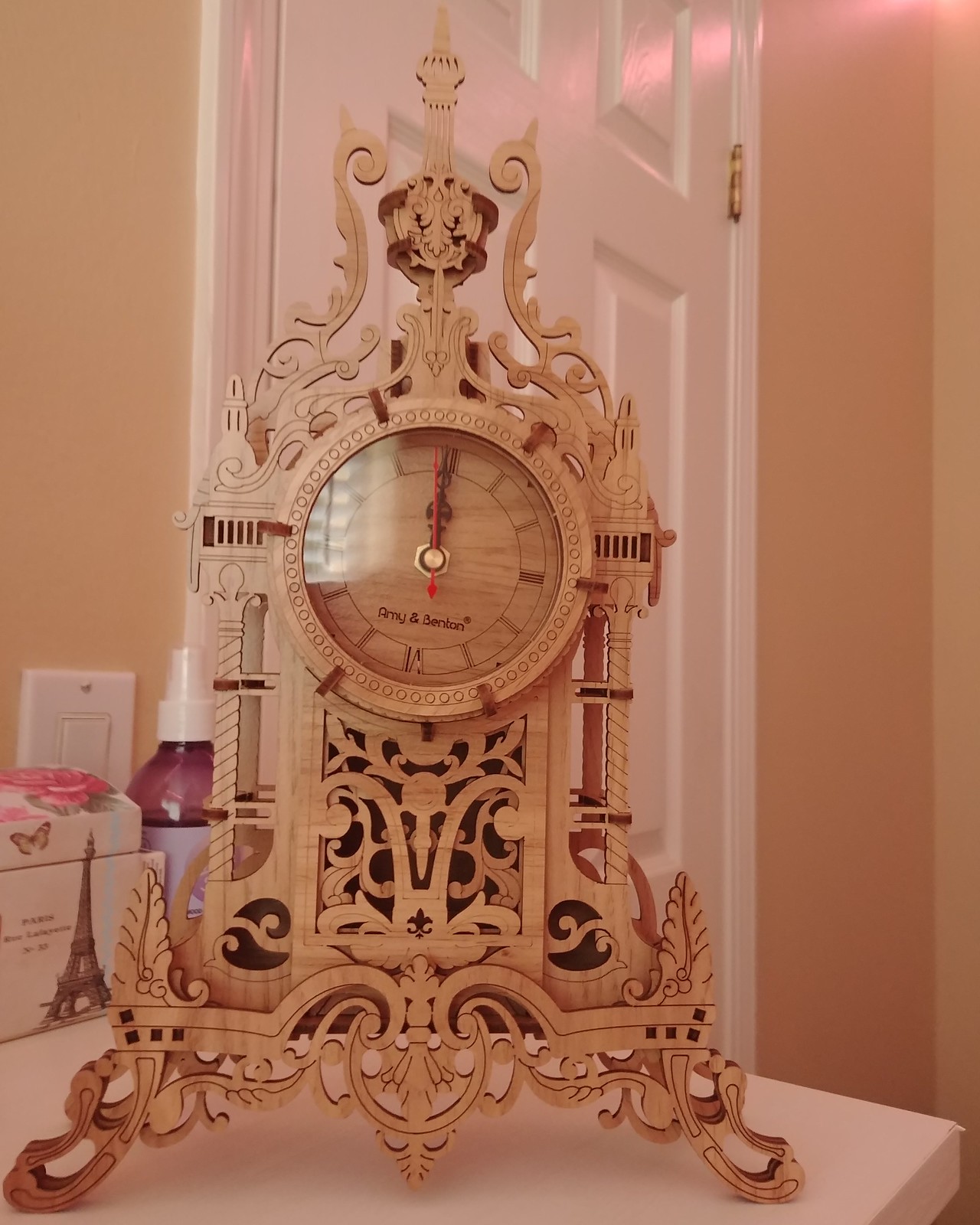The image showcases an ornate, intricately carved wooden clock, likely crafted from light-colored wood. The round clock face features Roman numerals, with both hands pointing to 12 and a red second hand also positioned at 12. Below the hands, a small strip of darker brown text reads "Amy and Benton." The casing of the clock is remarkably detailed with symmetrical curlicues, spirals, and peak structures that converge at the top, evoking an Art Deco style. The base of the clock is wider and features an etched rectangular cut-out adorned with curlicues, vines, and fleur-de-lis carvings, flanked by two small carved pillars.

The clock is displayed on a white shelf or desk against a pale peach wall and a white enamel-painted door. Additional items visible on the desk include a jewelry box with the Eiffel Tower, roses, and a butterfly design, as well as a spray bottle containing some liquid, possibly perfume. The setting, reminiscent of a bedroom, highlights the clock's elaborate craftsmanship and regal appearance.